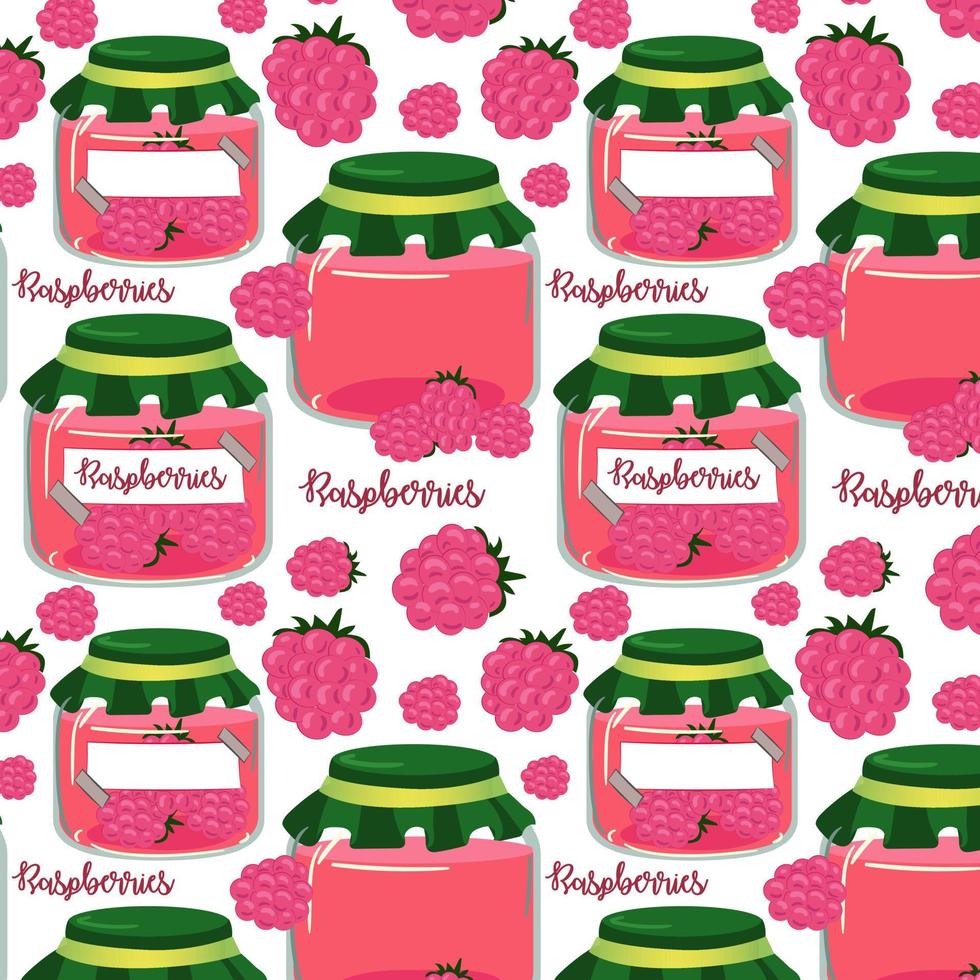This digital art image features a repeating pattern that prominently showcases jars of raspberry jam and fresh raspberries. The jars, made of transparent glass, have a cylindrical base and are topped with green, cloth-covered lids secured by light green rubber bands. Each jar contains a pink liquid, likely depicting the jam, and many of them display a label with the word "raspberries" and an illustration of raspberries. Some jars, however, either lack the label entirely or have an empty label. Scattered between these jars are depictions of pink raspberries, varying in size, some with green leaves on top. This intricate and repeating pattern, set against a clean white background, evokes the sense that it could be used for a tablecloth, wallpaper, quilt, or blanket, all designed to draw attention to and celebrate raspberries.